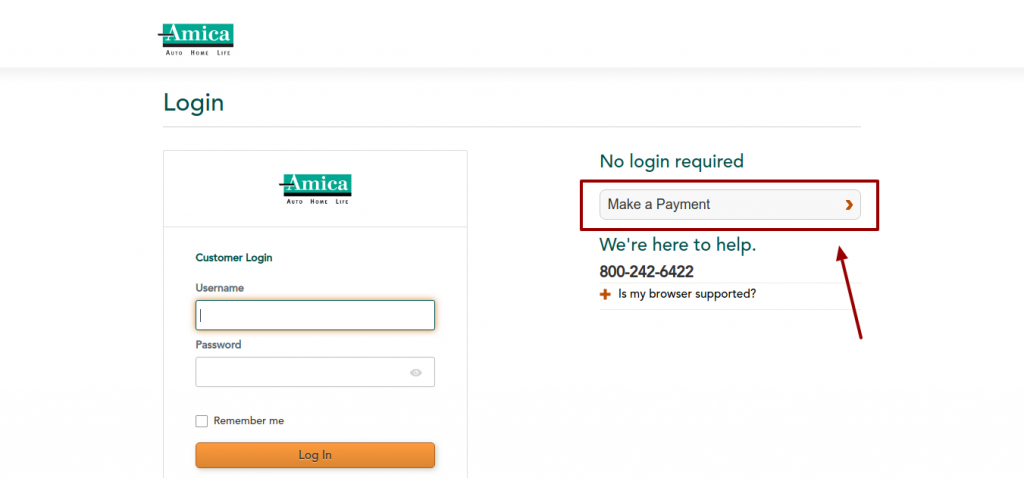On a white background, the upper left corner features the word "AMICA" in white font on a green background, followed by "Auto, Home, Life" also in white font on green. Below this, the text "Auto, Home, Life" is repeated in black on a white background. A gray line separates this header from the rest of the content.

Underneath the header, there is another section displaying the word "Login" in green, followed by another gray line. Repeating "AMICA" and "America" introduces the next section, with "Customer Login" prominently displayed below.

The login area includes fields for "Username" and "Password," both empty. A checkbox labeled "Remember Me" is present but not selected. The "Login" button, which is orange, is below these fields.

To the right, the text "No Login Required" introduces a button labeled "Make a Payment." This button is outlined in red, with a red right arrow next to the text.

The footer of the image provides assistance information, stating "We're here to help 800-242-6422," followed by "Is this supported in my browser?" in smaller text. The predominant colors in this layout include green, orange, red, white, black, and gray.